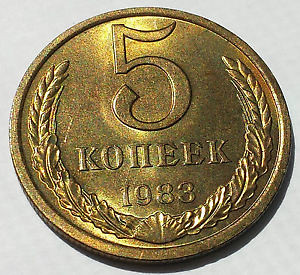The photograph showcases a shiny, brand-new looking coin with a golden, brassy hue, set against a textured white background, possibly a paper towel. Dominating the upper portion of the coin is a large, bold number "5," centrally positioned. Below this prominent numeral is the text, likely in Russian or Eastern European script, reading "KОИИEEK." Beneath the text, the year "1983" is clearly inscribed. A decorative pattern adorns the lower half of the coin, featuring two olive branches that extend upward towards the upper left and right edges, joined at the base by a scallop shell motif. The coin's edge is raised, providing a bezel-like appearance, and the photograph is slightly angled, showing the edge thickness, particularly at the bottom.